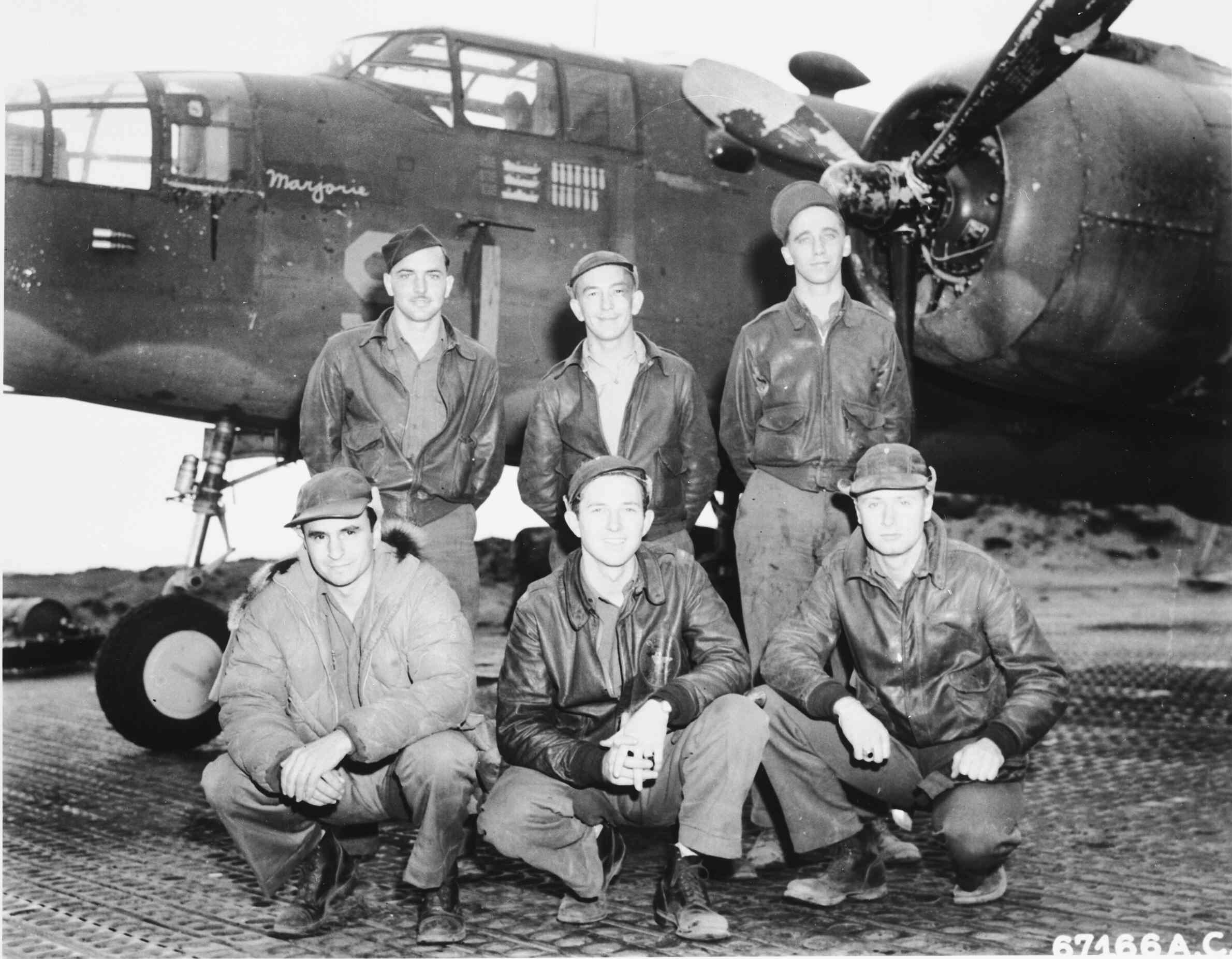This black and white antique photograph captures a group portrait of six white men proudly posing in front of an old-fashioned fighter-style aircraft named "Marjorie." The men are all dressed in neat leather jackets, boots, and what resemble newspaper boy caps. Their complexions appear particularly pale, likely due to the age of the photo, which renders the background somewhat washed out. Three men are crouched down in the front row while the remaining three stand behind them with their hands behind their backs. The backdrop features low-lying hills and a runway. In the bottom right-hand corner of the image, the label "67166AC" is visible, though slightly chopped off at the bottom. The overall scene is one of camaraderie and pride, capturing a moment in time of these aviators and their aircraft.